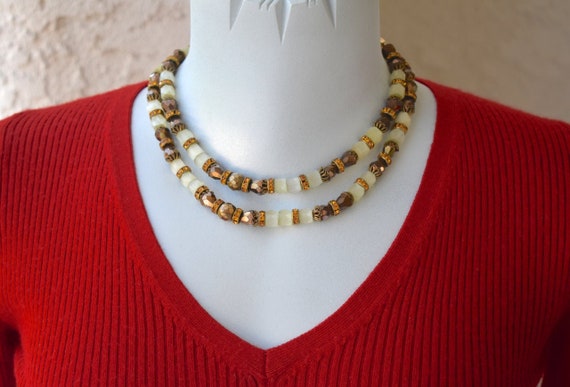The photograph features the upper chest and shoulders of a white plastic female mannequin, positioned against a textured, cream-colored stucco wall. The mannequin is adorned in a finely knit, red V-neck sweater with vertical ribbing, suggesting a lightweight material suitable for fall or spring. Around its neck, the mannequin wears a double-stranded necklace composed of a variety of beads, including clear whitish beads, and various shades of brown, gold, and rose-gold beads. The beads resemble small peas and alternate in size and color, adding a rich, detailed aesthetic to the ensemble. The necklace wraps around the neck twice, creating two visible cords, and appears to have a clasp at the back, though it is not visible in the photo. The overall composition appears to emphasize the detailed craftsmanship of the jewelry, possibly suggesting that the necklace is the featured item for sale or display.